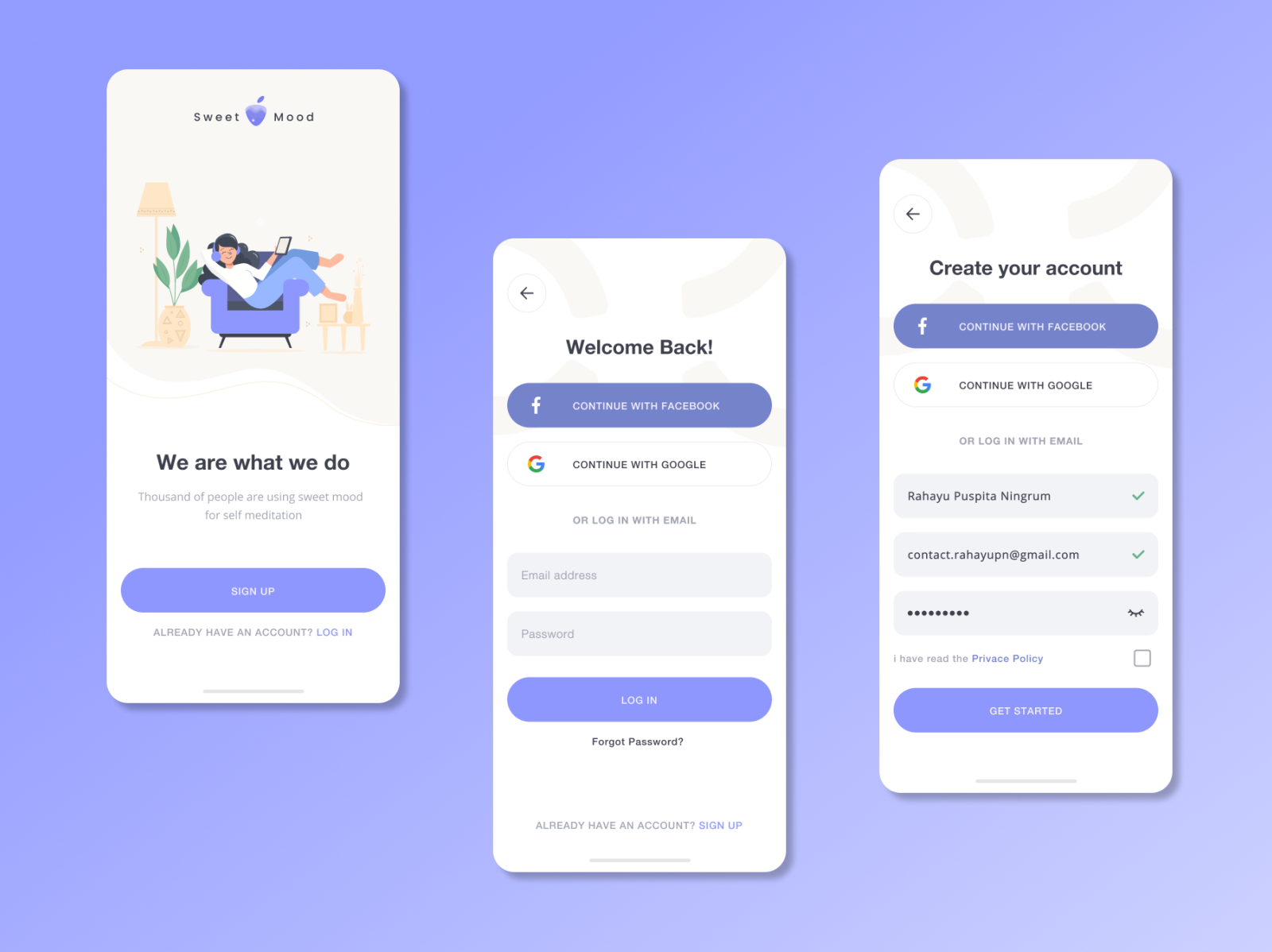This image showcases the Sweet Mood app, presented in a visually appealing layout with three different snippets displayed from left to right. The background transitions smoothly from a dark lavender at the top to a very light lavender at the bottom, creating a soothing gradient effect.

On the left side, "Sweet" is written next to an icon resembling an apple in the same dark lavender color. "Mood" is written in black, forming the title "Sweet Mood." Below the title, there's an image of an emoji depicting a woman lounging on a lavender loveseat. The woman has black hair and is dressed in light lavender pants while holding a tablet. Flanking the loveseat, a brown lamp and planter with a green plant add a touch of nature to the scene. To the right, a light brown end table holds a couple of objects, contributing to the cozy setting.

Beneath this, the text reads: "We are what we do. Thousands of people are using Sweet Mood for self-meditation." Following this message is a lavender button labeled "Sign Up." Directly below, a prompt for existing users states, "Already have an account? Log in," with "Login" highlighted in purple.

Further down, the text "Welcome back" appears above a purple button labeled "Continue with Facebook." Below this, a white button offers the option to "Continue with Google" or "Log in with email." Email address and password fields are ready to be filled in, presented within a gray bar. Below these fields, a purple button states "Log In," accompanied by options "Forgot Password?" and "Already have an account? Sign Up" in purple text.

To the right, users are invited to "Create your account," with fields for email address, name, and password already filled out. A purple button at the bottom encourages users to "Get Started."